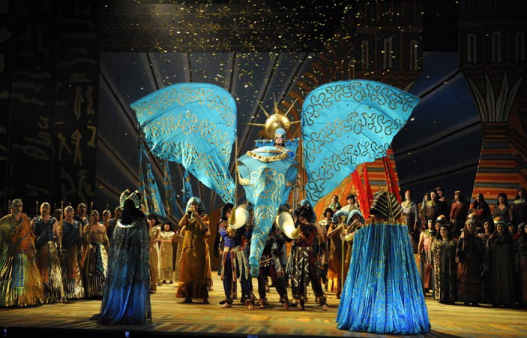The image depicts a visually striking scene of a theatrical or ceremonial gathering, possibly set in a dark, outdoor environment or on a dimly lit stage. Central to the composition is a large, fabricated blue elephant adorned with intricate gold patterns and flanked by man-made wings. A woman, dressed in elaborate, ancient Egyptian-inspired attire, is riding the elephant. The stage background features striped structures in red and gray, with hints of hieroglyphics on the back left, contributing to an ambiance reminiscent of an Egyptian tomb. The floor is a mix of brown and yellow hues. Surrounding the central figure are approximately 20 to 30 participants, all clad in a variety of culturally ornate costumes, predominantly in shades of blue, lending a cohesive color theme. These individuals, arranged in lines and clusters, wear long robes and headdresses that evoke the regality of an ancient royal court, albeit with a distinctive modern twist.